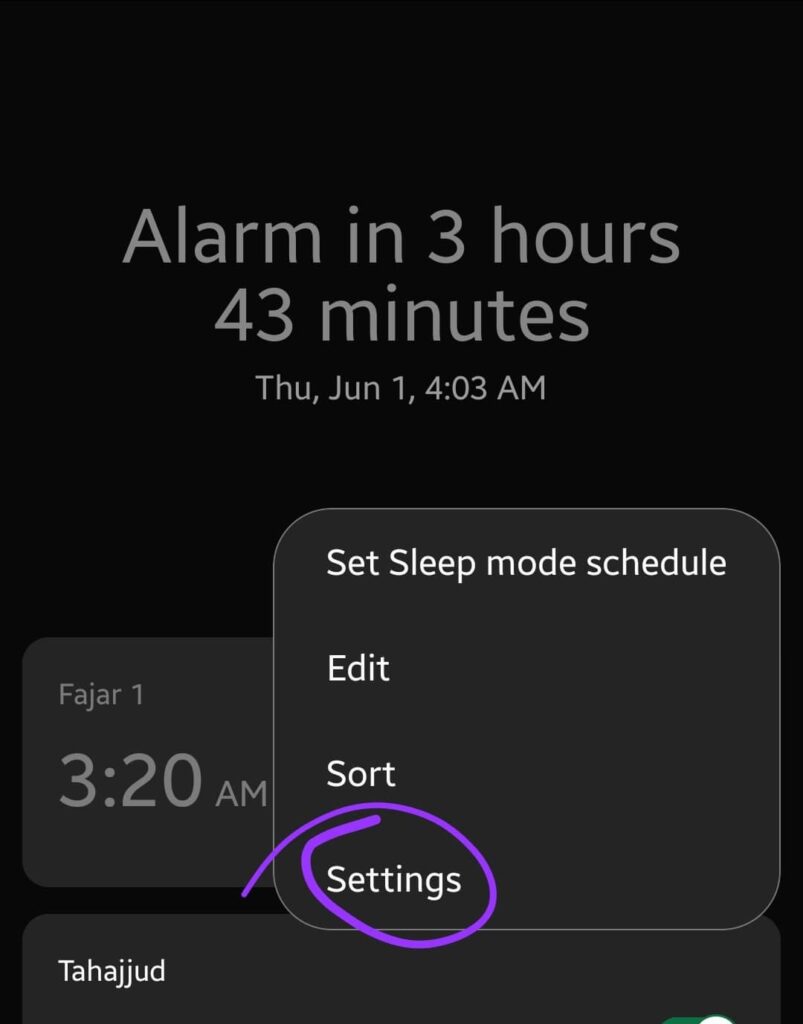A screenshot showcases a mobile alarm setting interface with a prominently featured alarm scheduled for 3 hours and 43 minutes from now. The current date displayed is Thursday, either January or June 1st, at 4:03 a.m. The interface reveals options to set up a sleep mode schedule just below the alarm time. A purple hand-drawn circle focuses attention on the ‘Settings’ option in this section. On the left is an entry labeled "Fajar" in small text, set for 3:20 a.m., with another entry beneath it called "Tahajud" in a different language. This entry has a slider button partially visible at the bottom right. The interface features a sleek design with a black background and white text, with the exception of the settings label, which is highlighted in color for emphasis.